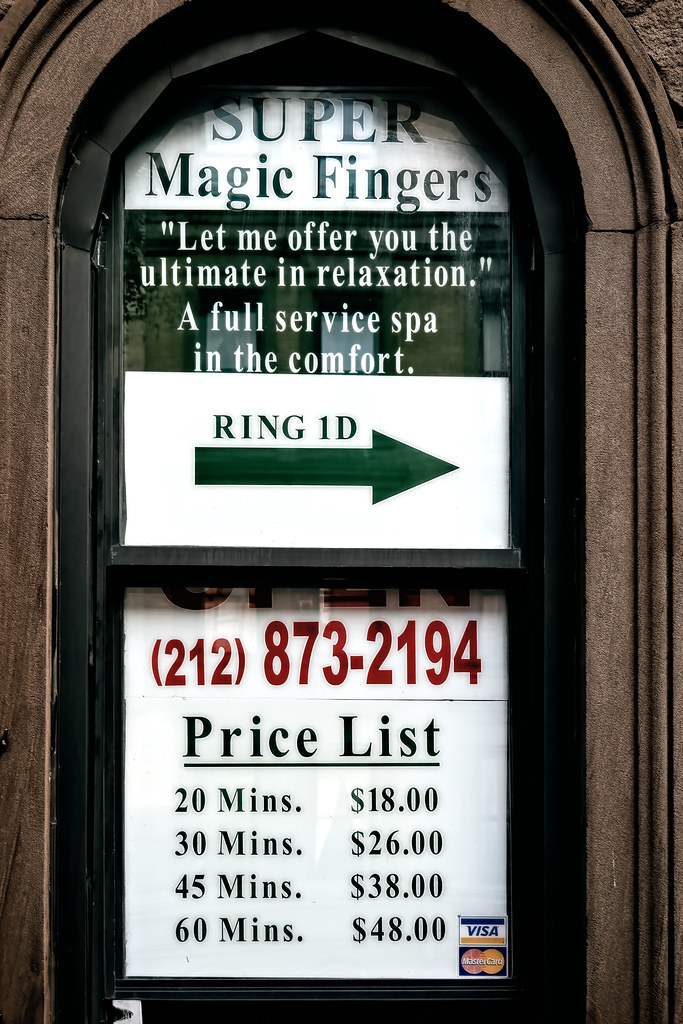The image is a colored daylight outdoor photograph showcasing the window of a business called "Super Magic Fingers." The window, framed by dark brown stone or wood, is divided into two sections by a black window frame. At the top of the window, a white sign with black text prominently displays the business name, "Super Magic Fingers." Below this, white text applied directly to the glass reads, "Let me offer you the ultimate in relaxation. A full-service spa in the comfort." Further down, there is a white sign with a green arrow pointing to the right, accompanied by green text that says "Ring 1D." Below this, on the lower half of the window, is a red phone number, "212-873-2194," followed by a price list in black text: $18 for 20 minutes, $26 for 30 minutes, $38 for 45 minutes, and $48 for 60 minutes. At the bottom right of the window, Visa and MasterCard logos are displayed. The overall setting indicates an exterior view, with the signage serving as an advertisement for the spa services offered inside.